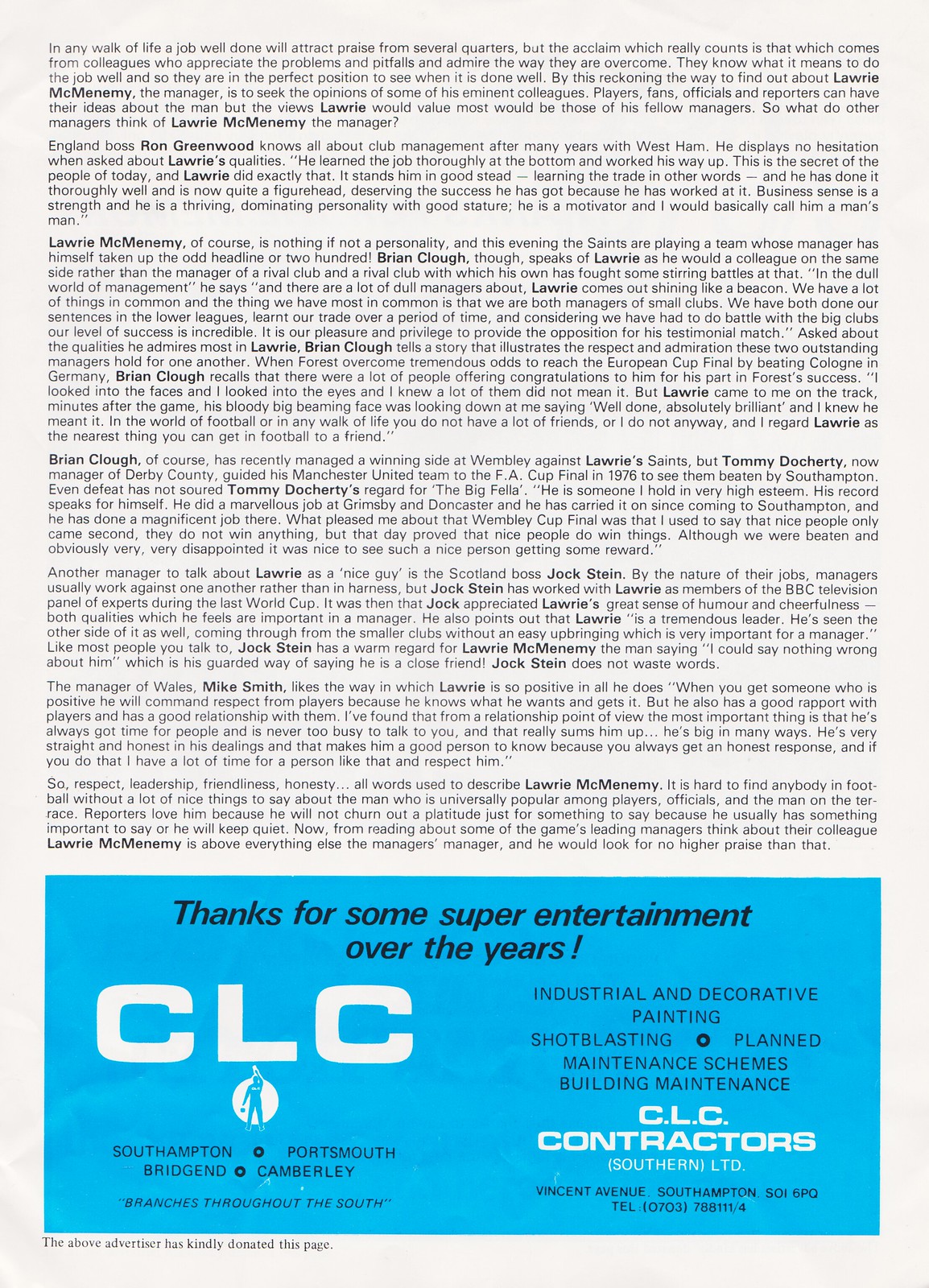This image features a black-and-white page from a magazine or newspaper, filled with dense black text detailing what seems to be a sports-related article with at least seven paragraphs. Key terms like "manager" and "Wembley Cup" are highlighted, suggesting a focus on sports events and figures. At the bottom of the page, there is a prominent blue rectangle containing an advertisement from CLC Contractors Southern Limited, thanking readers "for some super entertainment over the years!" The ad, highlighting their various services such as industrial and decorative painting, shop blasting, and planned maintenance schemes, lists their branches in Southampton, Portsmouth, Bridgend, and Camberley, with the main office located at Vincent Avenue, Southampton, SO15 5PO, including a contact telephone number. The ad also notes the company's generosity in donating the space for the advertisement.